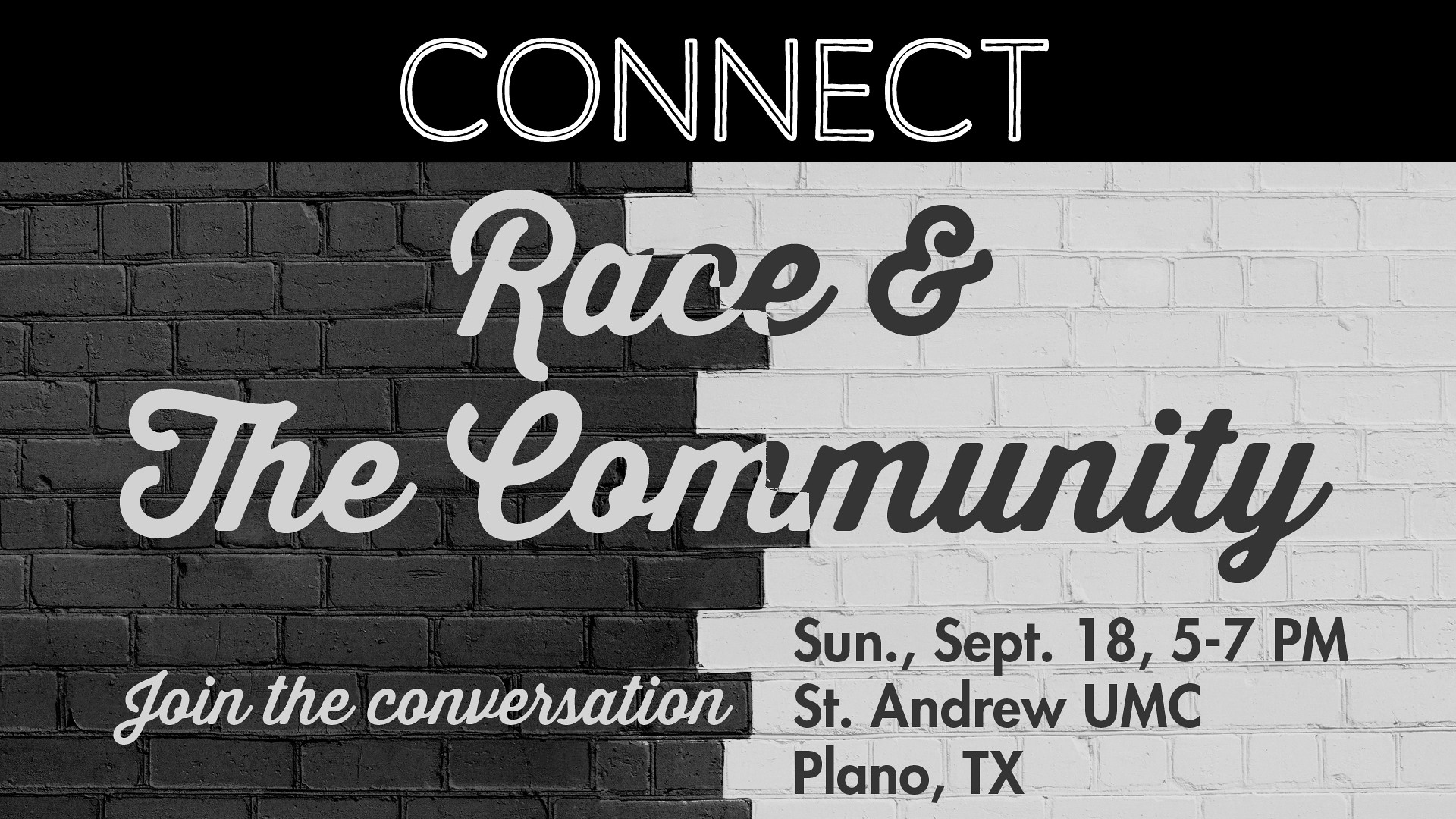The image showcases a rectangular sign with a predominantly white, black, and gray color scheme. At the top, a black rectangle with white capital letters spells out "CONNECT." Below this, the lower portion of the sign features a depiction of a brick wall. The left side of the wall is painted gray, while the right side is painted white. The bricks are unevenly oriented and alternate at different intervals. In cursive script, the words "RACE AND THE COMMUNITY" are written across the center. On the lower left in cursive, it states "JOIN THE CONVERSATION," while the lower right side provides event details: "SUNDAY, SEPTEMBER 18th, 5-7 p.m., St. Andrew, UMC, Plano, Texas."